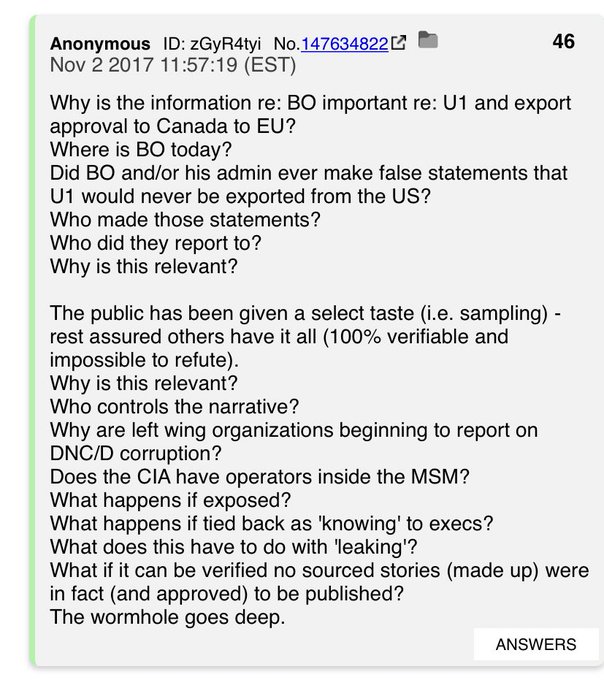This image is a screenshot of a 4chan post, characterized by its distinctive layout. At the top left corner, a gray section with the label "Anonymous" identifies the poster. Adjacent to this, in bold black print, is the user ID, followed by the message number, which is underlined in blue and displayed in blue numerals. To the right of the message number are two icons: a share icon, and a gray folder icon.

On the far left, the number "46" is indicated in black. Below this, the post begins, revealing a lengthy and somewhat disjointed message. The content of the message includes questions probing the importance of information related to REBO, the export approval processes involving Canada and the EU, and inquiries about "BO," likely referring to Barack Obama. The message queries whether Barack Obama or his administration ever falsely claimed that U1, presumably Uranium One, would not be exported from the U.S., and seeks information on who made such statements and to whom they reported. The relevance of these claims is also questioned.

The post continues with additional rambling commentary. In the bottom right corner of the screenshot, a white box labeled "Answers for replies" is present, presumably for users to respond to the post.